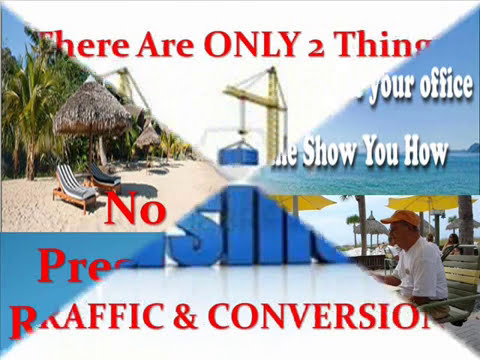This image is a strange, collage-like advertisement that combines multiple advertisements into one disjointed visual. The wide rectangular graphic resembles a screenshot from a PowerPoint presentation and is segmented into six triangles—three main sections, each further divided on the left and right, resulting from diagonal cuts. Dominating the top triangle with a white background, red text proclaims "there are only two things," and features an image of a yellow crane. The lower triangle emphasizes "traffic and conversion" against a backdrop of tall blue letters. On the left side, a beach scene showcases palm trees, a hut, and chairs under the sun, with the words "no" and fragments of other text visible in red font over a blue background. The right side contains an image of a man sitting on a wooden swing, partially under an umbrella in a lawn chair, coupled with phrases like "your office me show you how." The colors spanning the image include black, white, gray, yellow, orange, red, green, and various shades of blue, adding to the visual chaos and eclectic mixture of elements. The overall composition makes it challenging to discern a cohesive context, as it is essentially a patchwork of different cutouts and motifs pasted together.